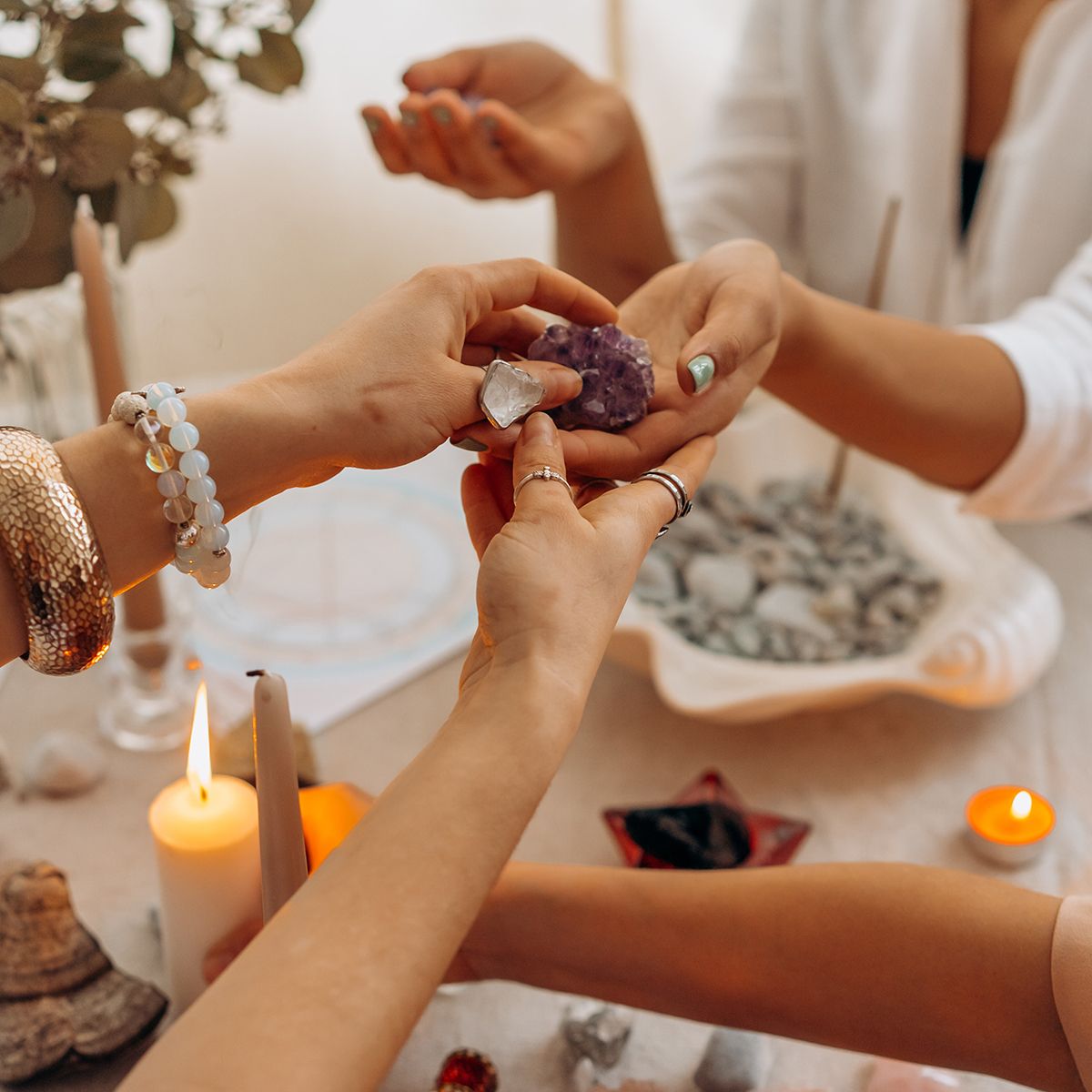The photograph captures an intimate scene centered around a transaction of a purple gemstone, potentially amethyst, between a few women whose faces are not visible. The focal point is on their hands and partial upper bodies. One woman, adorned with a variety of jewelry including beaded and gold cuff bracelets on her left wrist and rings on her right hand, is handing the gemstone to another woman whose hands are extended with palms up. This second woman is identifiable by her seafoam green painted nails and white shirt. A third person, whose body is mostly obscured, reaches over with a lit candle from the left side of the image. They are positioned over a white table decorated with various objects including two or three lit candles, another unlit and taller candle in the background, and a plant. The background appears blurred, keeping the attention on the delicate exchange and the atmospheric candlelight.